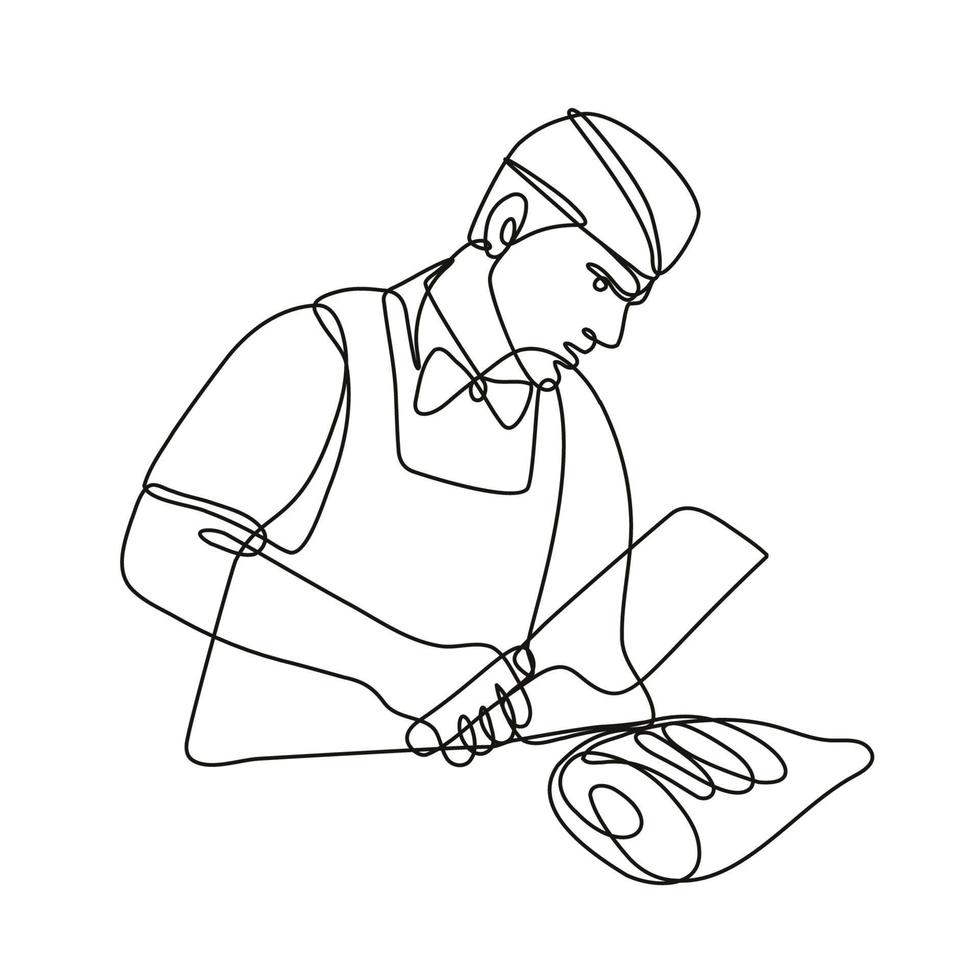This is a stylized, continuous black line drawing that resembles a neon sign with no breaks in the lines. The illustration depicts a man, likely a butcher or a chef, poised to cut into a piece of meat on a chopping board with a large meat cleaver. He wears a head covering, a bow tie, an apron, and a short-sleeved shirt, and his eyes are focused downward on the task at hand. The background is white, accentuating the simplicity and clarity of the black lines. The detailed depiction includes squiggly lines that form the uninterrupted outline of the butcher, emphasizing his attire and the meat-cutting action. The sketch has a computer-generated appearance, lacking an artist's signature, and suggests a utilitarian purpose such as an illustration in a book or an advertisement.